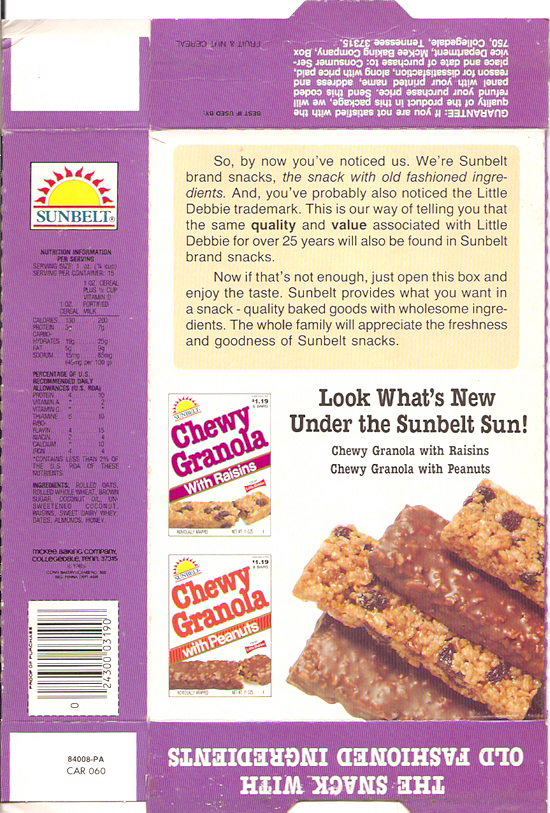This detailed photograph captures the back of a opened and flattened cardboard box that originally packaged granola products. The box is primarily a purple color, and features several distinct elements. 

On the left side of the image, there are smaller images of product boxes with the label "Chewy Granola" prominently displayed in a burgundy red color and another label in an orange hue beneath it. These product images signify different varieties of granola, including some with raisins and others with peanuts.

The right side of the image showcases an assortment of granola bars, individually unwrapped with some of them partially covered in chocolate, highlighting the range of styles available.

At the top left corner of the box, the product logo "Sun Belt" is presented in an aqua color, accompanied by a graphic of a yellow sun with red rays, encased within a white rectangular area. Below this logo, you can find detailed information about the product, including nutritional facts and the vitamins and minerals it contains.

Toward the bottom of the box, there is a black barcode printed on a white background, providing additional product details necessary for retail purposes.